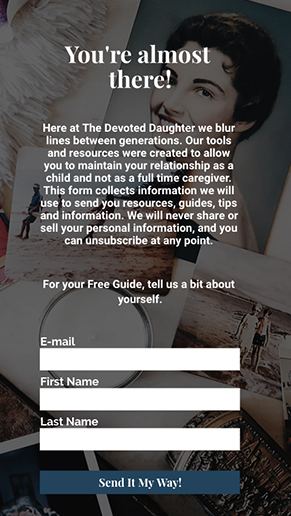The image features a visually striking canvas composed of various photographs. Dominating the top section is a semi-grayscale image of a white woman with flowing black hair and vibrant red lipstick, giving a vintage, noir-inspired aesthetic. Surrounding her photo are smaller, layered images depicting people by the ocean or at a beach, creating a layered tapestry of memories and moments.

In the center of this artistic assembly is a bold, prominent message that reads, "You're Almost There." Below this eye-catching heading, additional text in a clean, professional font reads: "Here at The Devoted Daughter, we blur lines between generations. Our chosen resources were created to allow you to maintain your relationship as a child and not as a full-time caregiver. This information collects information we use to send you resources, guides, tips, and information. We will never share or sell your personal information, and you can unsubscribe at any time. For your free guide, Tell Us A Bit About Yourself."

Underneath this paragraph are three input fields labeled "Email," "First Name," and "Last Name," each accompanied by a blank box ready for user entry. Concluding the layout is a call-to-action button with the text, "Send It My Way," inviting viewers to engage and receive further resources.